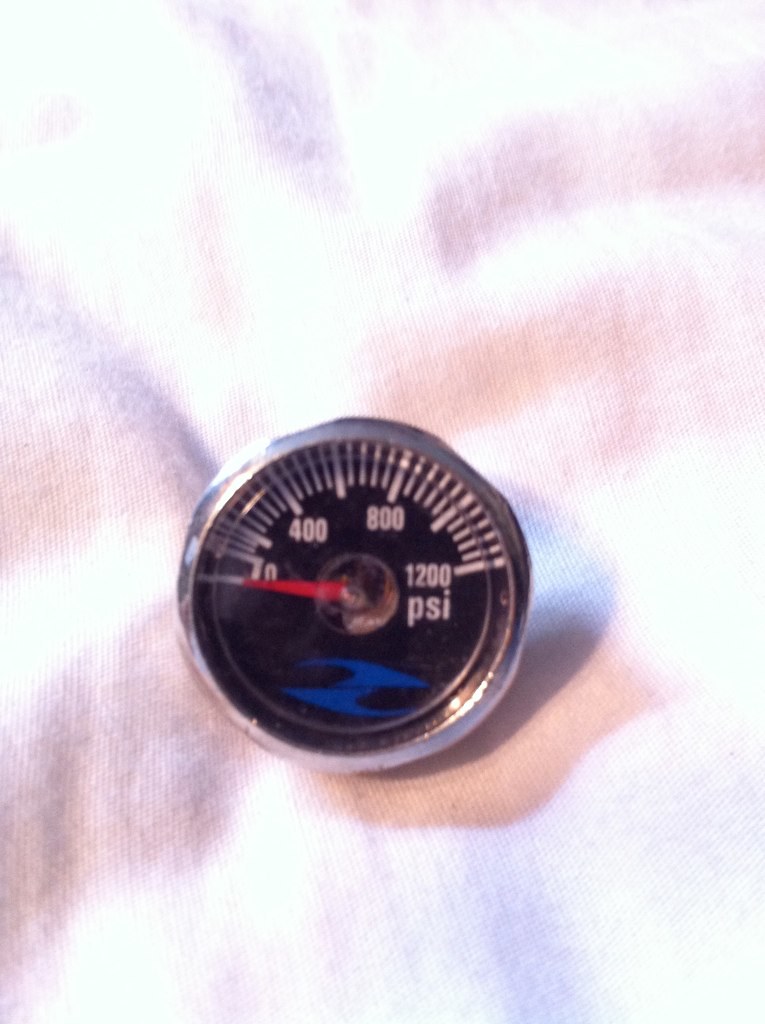This photograph features a visually complex background that transitions through various shades and colors. At the bottom, a muted gray tone sets the stage, intersected by a dark gray line ascending through the center. Above this, the backdrop showcases a mix of red hues blending into a shaded region. The scene then transforms into alternating bands of white and purple, culminating with purple at the very top and finishing with white.

Dominating the center of the composition is a prominent silver circle, likely a temperature or pressure gauge. Within this circle, the inner section features a black background highlighted by a subtle blue design at the bottom. The focal point of the gauge is a red needle or arm that indicates measurements, currently pointing to the left at zero. Surrounding the arm are gradations marked by lines and numerals: starting from zero, progressing to 400, 800, and finally 1200 PSI, with "PSI" clearly labeled below the final measurement. This intricate description encapsulates both the aesthetic and functional elements of the photograph.